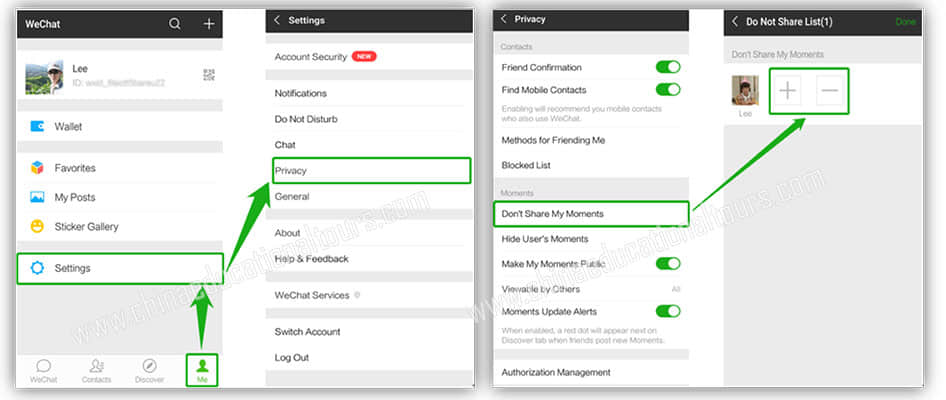**Descriptive Caption:**

The composite image consists of four horizontally aligned screenshots taken from the WeChat mobile app, depicting a step-by-step guide. Each screenshot is a distinct step in the tutorial, with elements highlighted for clarity. The entire image is overlaid with a semi-transparent watermark reading "www.chimaod.com," repeated diagonally twice.

1. **First Screenshot: Main Menu**
   - The screenshot features the main "Me" section in WeChat, with a black navigation bar at the top.
   - Prominent user details such as the user's name, "Lee," and avatar are displayed.
   - Key menus include Wallet, Favorites, My Photos, Sticker Gallery, and Settings.
   - The Settings option is encircled with a green rounded rectangle highlighted by an arrow, indicating it's the first step.
   - Navigation icons at the bottom of the screen include WeChat, Contacts, Discover, and Me, with "Me" similarly highlighted.

2. **Second Screenshot: Settings Menu**
   - This screen displays the Settings menu with a series of options: Account Security, Notifications, Do Not Disturb, and Privacy.
   - The Privacy option is highlighted with a green border and an arrow, indicating it's the focus of this step.

3. **Third Screenshot: Privacy Menu**
   - This menu showcases various privacy settings, with blue toggle switches for options such as Friend Confirmation and Find Mobile Contacts, both enabled.
   - The "Don't Share My Moments" toggle is particularly accentuated with a green outline, though without an arrow this time.

4. **Fourth Screenshot: Do Not Share Moments**
   - The final screen emphasizes the "Do Not Share" option, with "Do Not Share" displayed in white text on a black bar at the top.
   - The "Done" button is highlighted in green, and below it is a grayed-out "Don't Share My Moments" section.
   - The highlighted section includes an avatar picture and plus/minus signs, indicating selectivity options for the user's Moments sharing, outlined in green with an arrow pointing to it.

This image provides a clear visual guide for navigating privacy settings in the WeChat app, evidenced by the strategically placed highlights and arrows in the sequence of steps from left to right.